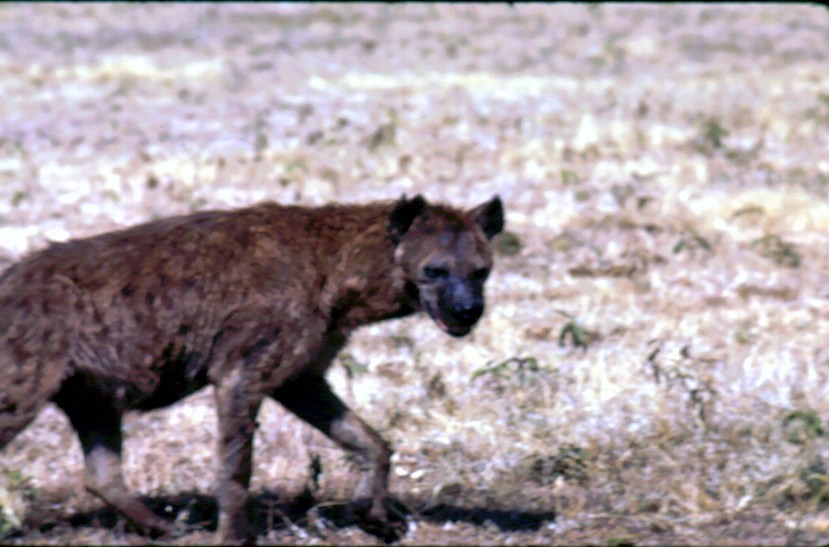The image depicts a dark brown hyena with a black snout, positioned in the lower left corner, growling while walking through a dry, arid field under bright daylight. The hyena, the sole subject of the photo, appears to be aware of the camera, its gaze directed towards it, adding a sense of immediacy to the scene. The three visible legs suggest movement, while the absent fourth leg contributes to a dynamic portrayal. The arid landscape, devoid of vegetation except for a few sparse, dry grasses and dead shrubs, forms a dull, grayish-white background that seamlessly blends with the hyena's coloring, emphasizing its presence. The photograph is a clear example of wildlife photography, capturing the raw, untamed essence of the wild in a vivid, yet desolate setting.